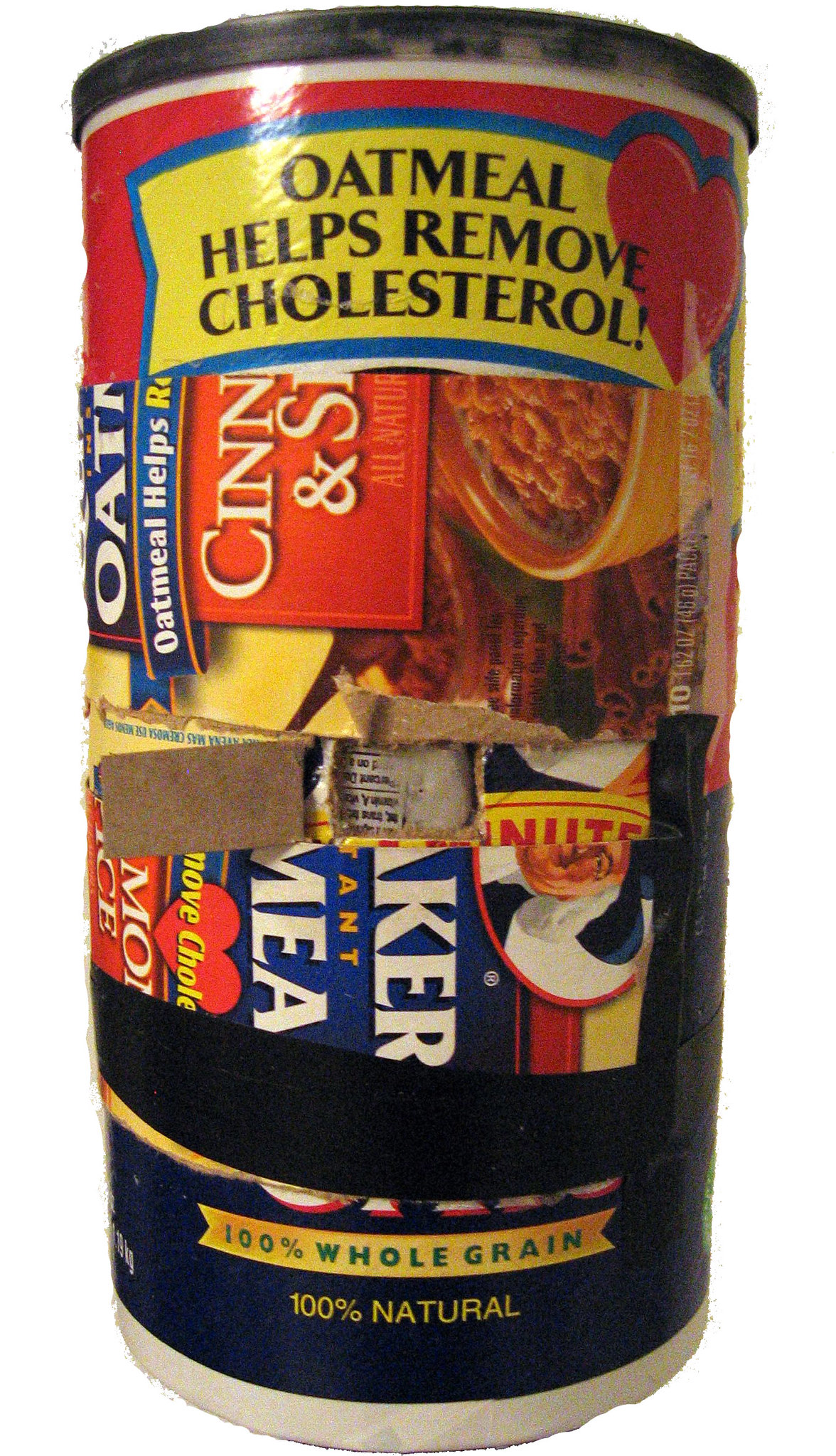The image showcases a slightly taller-than-wide cardboard canister against a solid white background that seamlessly blends into its surrounding area. This old-fashioned cylindrical container, reminiscent of those large oatmeal packages, has been creatively patched together using several horizontal labels and stickers from different oatmeal products. The top portion prominently features a yellow label with black text reading "Oatmeal Helps Remove Cholesterol." Below it, various overlapping and partially ripped labels display names such as Quaker Oats, with mentions of flavors like cinnamon and sugar, indicating processed oatmeal types. The original dark blue label at the bottom proudly states "100% Whole Grain" and "100% Natural." The assortment of labels suggests a history of diverse oatmeal consumption, pieced together, possibly in a bid to stabilize the canister and prevent its contents from spilling. Each label contributes to a collage effect, creating an eclectic yet cohesive visual of different oatmeal brands and types on a single container.